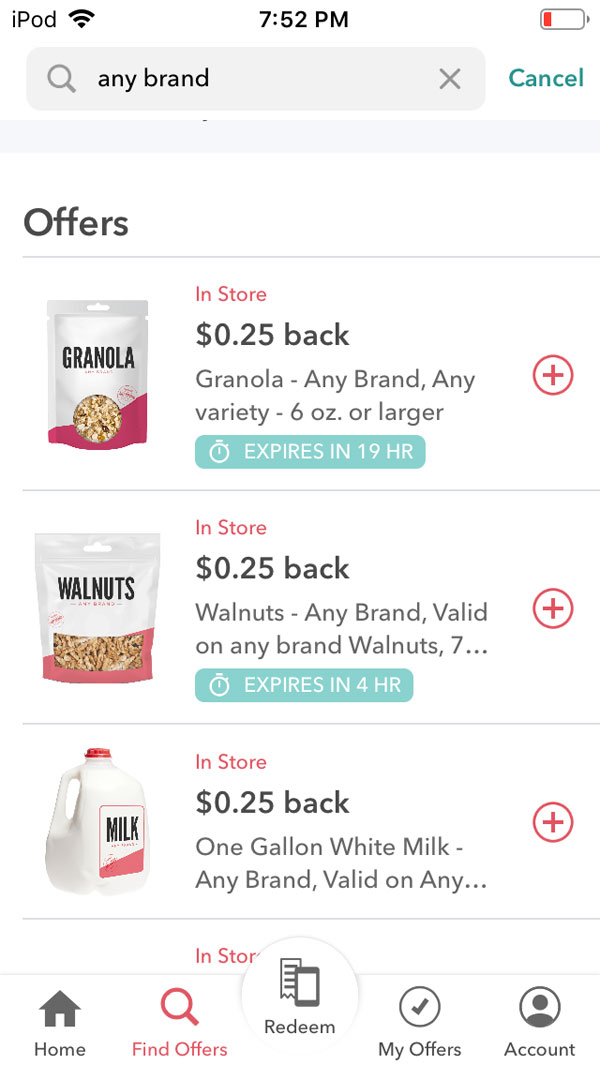The image depicts a user interface on an iPod screen, showing the time at 7:52 PM with a nearly depleted battery indicated. At the top of the screen, there's a search box labeled "Any Brand," featuring a magnifying glass icon and an 'X' for clearing the search, with a "Cancel" button on the right side.

Below the search box, the screen displays various offers. The first offer is for a bag of granola, depicted in a white and purple package, with the text: "In-store: 25 cents back on granola, any brand, any variety, 6 ounces or larger." This offer includes a circle with a plus sign and a blue box noting that it "expires in 19 hours."

Following this is another offer for a bag of walnuts, also in a white and purple package, with the text: "In-store: 25 cents back on walnuts, any brand, valid on any brand walnuts 7...". This too features a circle with a plus sign.

The final offer shown is for a gallon of white milk, with text: "In-store: 25 cents back on one gallon white milk, any brand, valid on any."